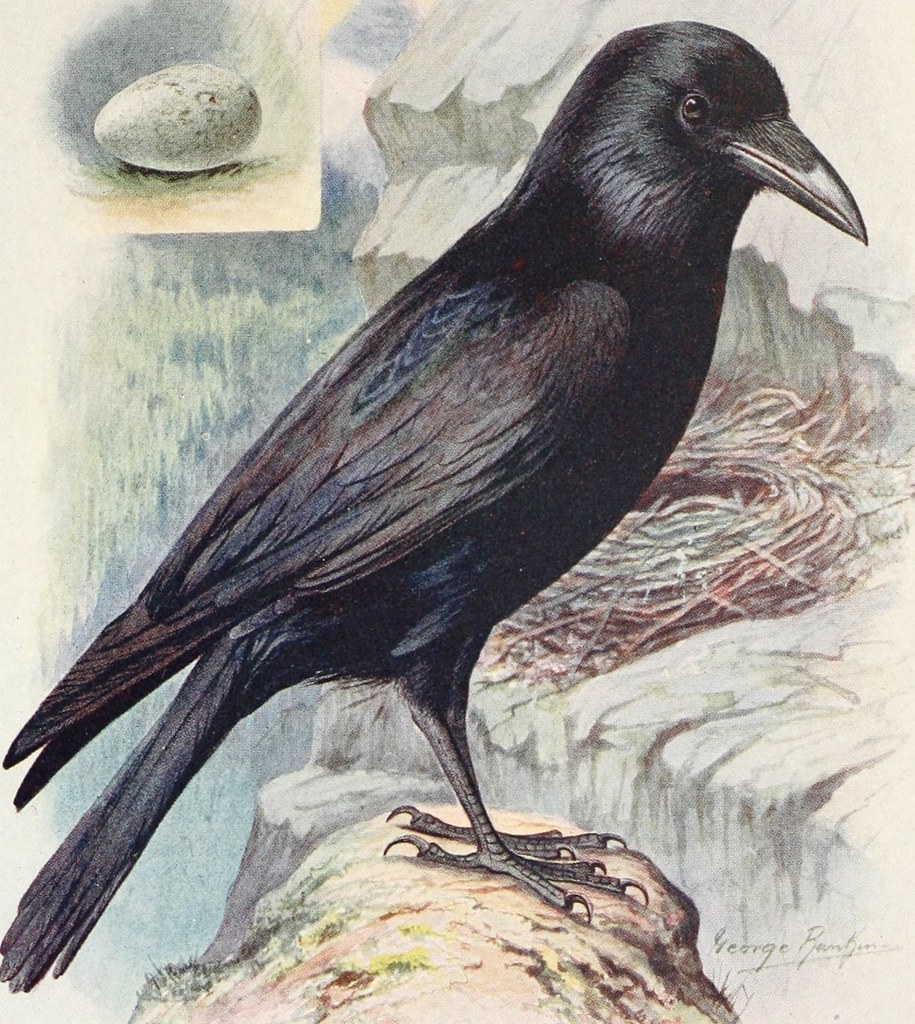The painting by George Rampkins features a detailed depiction of a black crow, some of its plumage tinged with gray and dark blue shades. The bird stands confidently on a small, multicolored rock that exhibits hues of gray, white, and tan. Behind the bird, a nest crafted from twigs is precariously perched on a rocky cliff face. The background reveals a mixture of green, white, and gray elements, possibly representing trees or bushes. In the upper left corner of the canvas, an inset image of the crow’s egg is visible. The egg is white with distinctive black or brown specks, set against a backdrop of blue and green grass with surrounding brown dirt. The bird's sharp black talons and pointed beak add further detail to the scene, while the artist's handwritten signature, "George Rampkins," graces the lower bottom corner of this intricate composition.